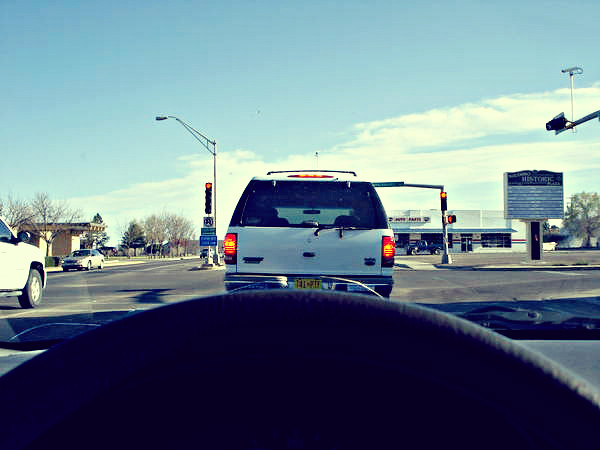A white Chevrolet Tahoe is positioned directly ahead of the vehicle from which the photo is taken. The Tahoe’s red taillights are illuminated, indicating either braking or stopping. The rear of the Tahoe features a large, clear, rectangular back window, through which the interior can be faintly seen. The vehicle also has a yellow rectangular license plate affixed to the bottom of its frame. In the foreground, the top of the black steering wheel and the gray dashboard of the photographer’s car are visible, along with the car's black hood. The scene unfolds on a dark gray paved road, bordered by several street lights and lamps made of gray metal. The sky above is a vivid blue, adorned with wispy, white clouds.